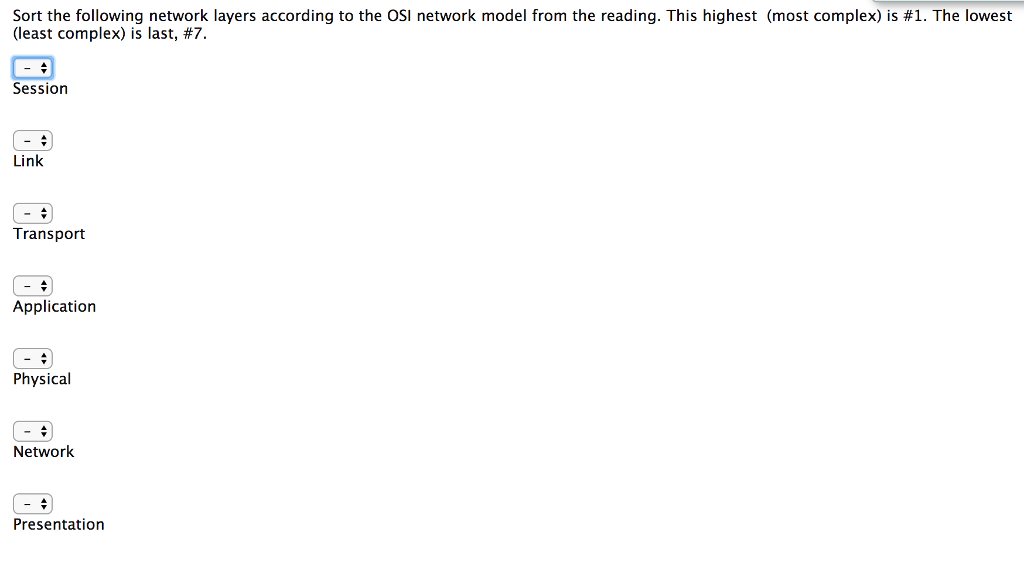**Detailed Caption:**

The image displays a predominantly white page that appears to be part of an app or a website, with a header section at the top that contains options not fully visible in the image. In the upper right-hand corner, there is the faint shadow of a button or a search field, indicating its presence without showing the actual element.

Below this, there's an instructional prompt which reads, "Sort the following network layers according to the OSI network model from the reading, the highest [most complex] is number one, the lowest [least complex] is last, number seven." Underneath this prompt are seven dropdown options, each paired with a corresponding network layer name. 

These dropdowns are currently unselected, signified by a rectangular button with up and down arrows that display a dashed line indicating no number has been chosen. The first dropdown is highlighted with a blue shadow, suggesting it is currently selected or focused.

The network layers listed in sequential order, from top to bottom, are:
1. Session
2. Link
3. Transport
4. Application
5. Physical
6. Network
7. Presentation

Each network layer name is paired with an unselected dropdown button beside it. The text alignment of the layers is justified to the left, and the rest of the page remains empty, without any additional text or elements.